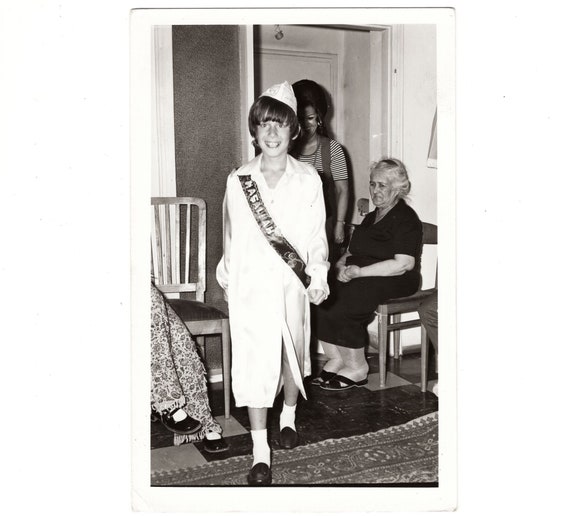This black-and-white photograph, framed with an eggshell white outline, captures a moment inside a family living room. Dominating the vertical rectangular frame, a child, possibly around 11 years old, stands prominently in the left center. The child is dressed in a long white graduation jacket, a black sash draped across it, and wears a white cap at a jaunty angle, grinning widely. The child’s attire is completed with white socks and black shoes. Just over the child's shoulder, a person with voluminous but short hair, clad in a dark and white striped t-shirt, follows closely, smiling menacingly at the camera. To the right, an elderly woman with silvery hair sits calmly in a chair, dressed in a simple black dress and black strapped shoes. The left side of the photograph shows the legs of another individual sitting on a wooden chair, wearing black shoes and floral patterned pants. The image beautifully encapsulates a familial scene with each person seemingly connected to the joyful occasion signified by the child's graduation attire.